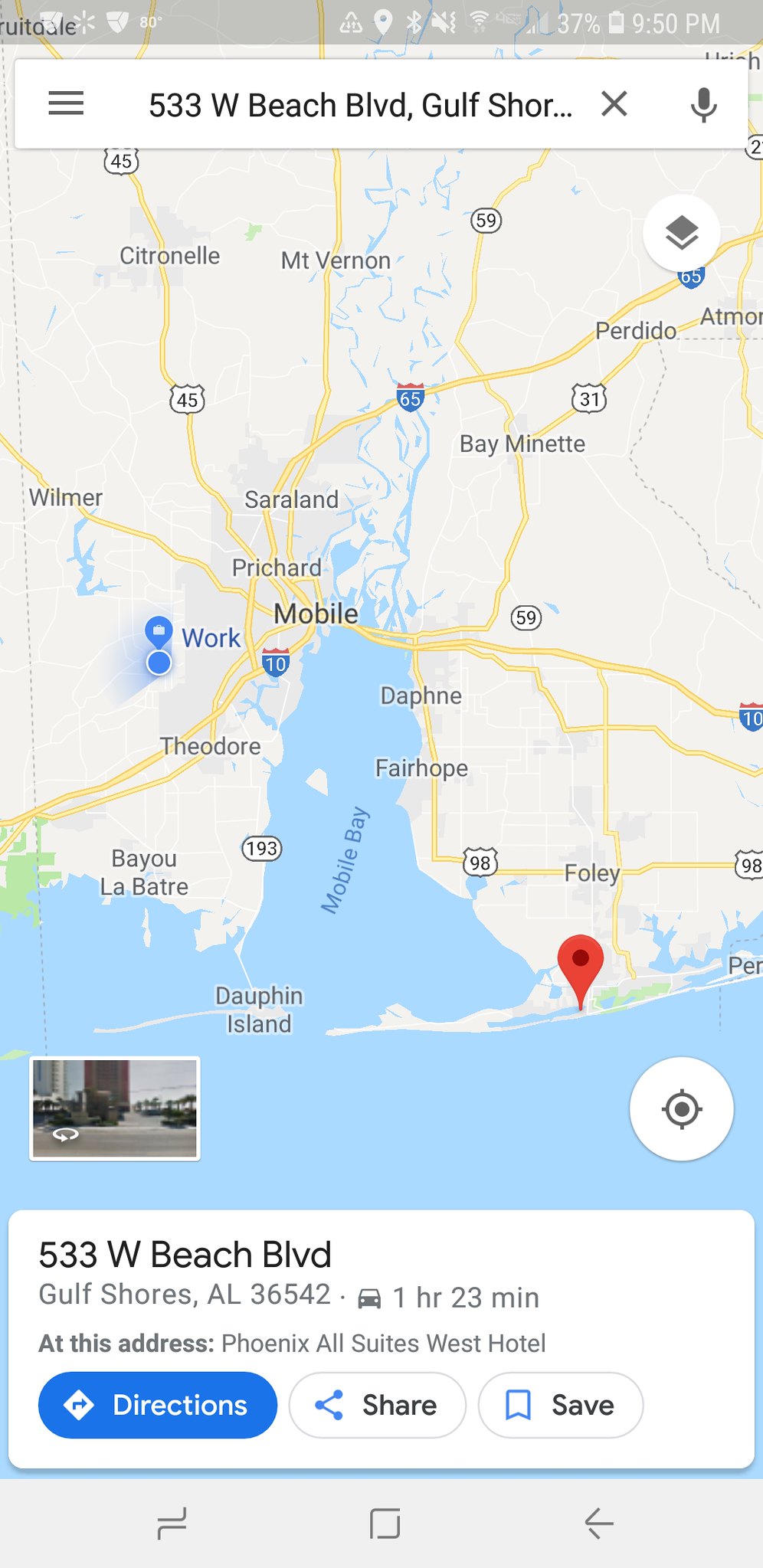The image depicts a detailed screenshot of a smartphone displaying a map centered on the Gulf Shores of Alabama, specifically highlighting the address 533 West Beach Boulevard. The phone's status bar at the top shows a battery percentage of 37% and the time, 9:50 PM, along with various icons such as the Wi-Fi signal. Below this, a search bar reflects the same address, accompanied by a microphone icon. The map features yellow lines for roads and highways, blue for water bodies like Mobile Bay, and off-white for land areas, with labels for several cities including Mobile, Fairhope, Daphne, Saraland, Bay Minette, and Mount Vernon. A notable blue dot indicates the user's workplace, while a red balloon pinpoints the specified address. On the left, there is a street view thumbnail, and just below it, a text box reiterates the address and shows an image of a car, indicating a travel time of 1 hour and 23 minutes to reach "Phoenix All Suites West Hotel" from the current location. Beneath the details, a blue banner offers “Directions”, and adjacent options to share or save the location.